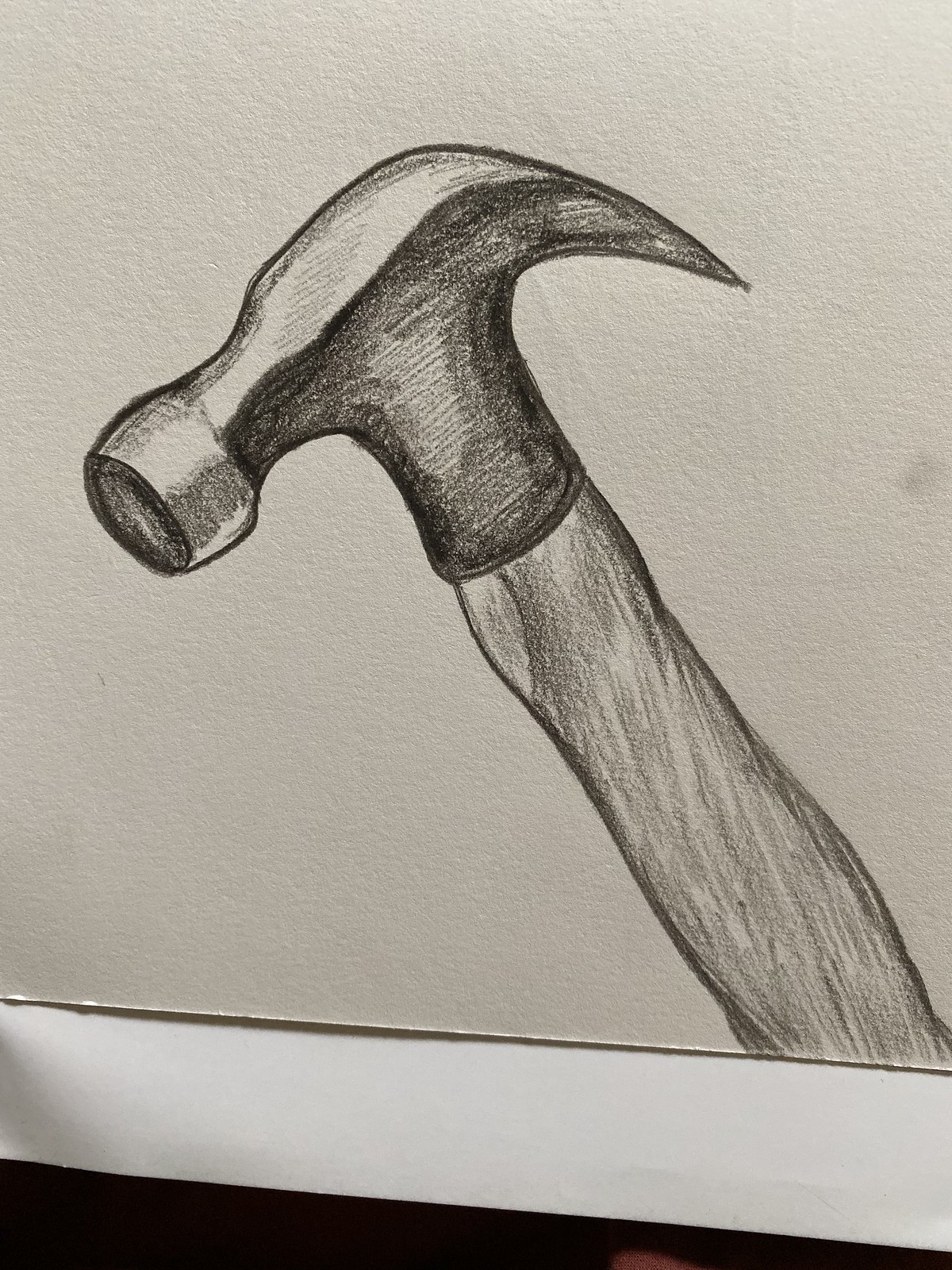The image depicts a detailed pencil sketch of a hammer, rendered with rich shading that enhances its realistic appearance. The hammer's head is depicted in a darker shade of black than the handle, which features angled curves likely intended to improve grip and dexterity. The artwork, drawn on a slightly beige piece of sketch paper, occupies about 60% of the image, with the hammer's face oriented towards the bottom right corner. Subtle highlights suggest light reflecting off the hammer, further accentuating its three-dimensional form. The sketch is placed on what appears to be a white tabletop or an easel, possibly indicated by hints of brown and darkness suggesting support structure. The background around the paper has a creamish tint, adding depth and context to the scene. Additionally, a small, indistinct object, possibly a finger, peeks from the bottom edge of the photo, lending a casual, in-progress feel to the artwork.